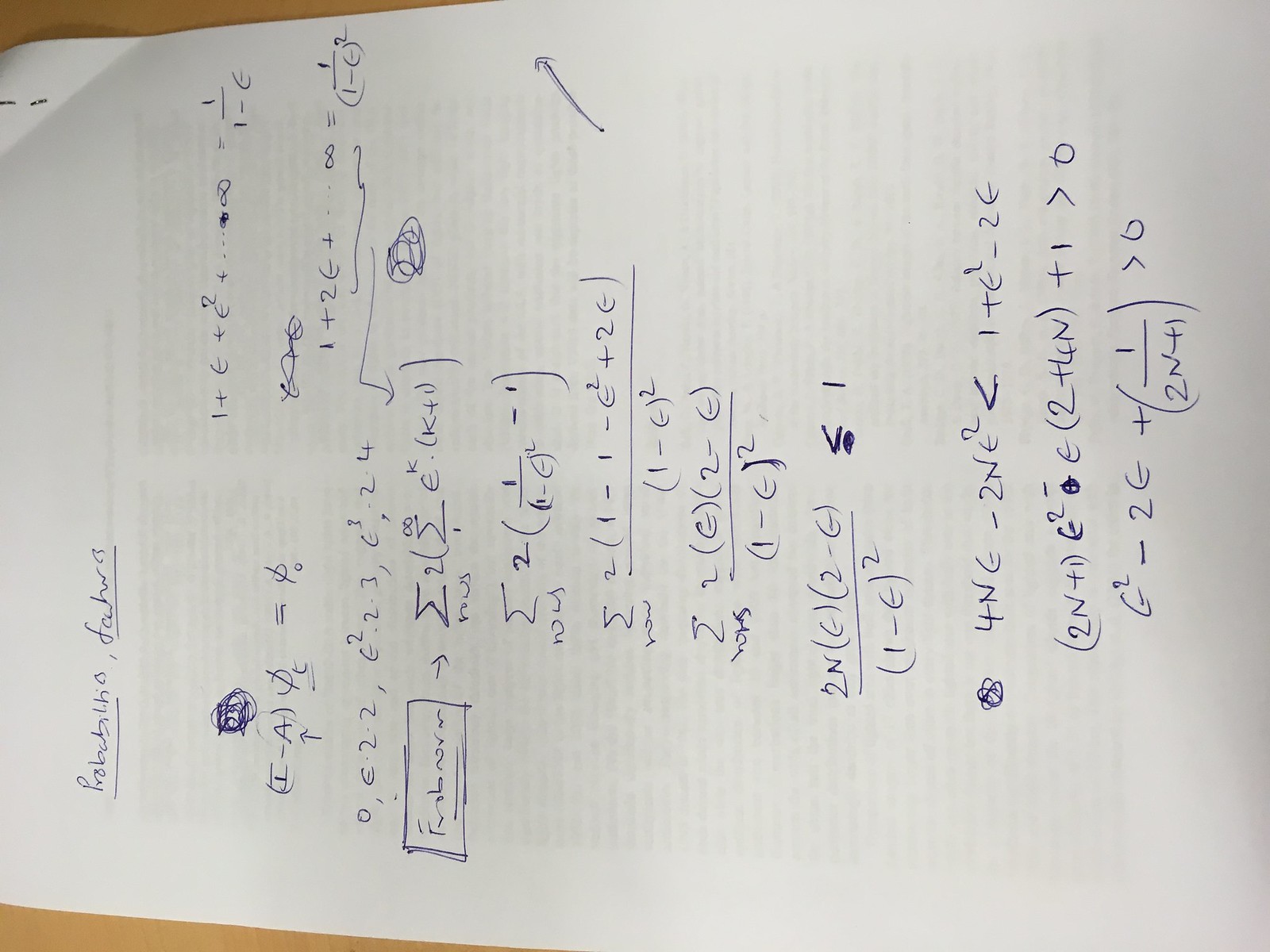This is a detailed color photograph of a piece of white paper, slightly tilted to the side, filled with intricate mathematical equations written in blue ballpoint pen. The equations feature a mix of letters and numbers, including symbols such as plus signs, parentheses, and what appears to be the Greek letter epsilon (ε). Some recognizable portions of the equations include "1 + 2 + ε + ... ∞ = 1 / (1 - ε^2)," and another sequence "4 - N - ε - 2Nε." There's a more complex part that reads, "ε^2 < 1 + ε^2 - 2ε." At the very bottom of the page, an equation is visible: "G^2 - 2G + (1 / 2N + 1) > 0." The series of equations suggests a detailed and thorough work on some advanced mathematical or physical problem-solving.